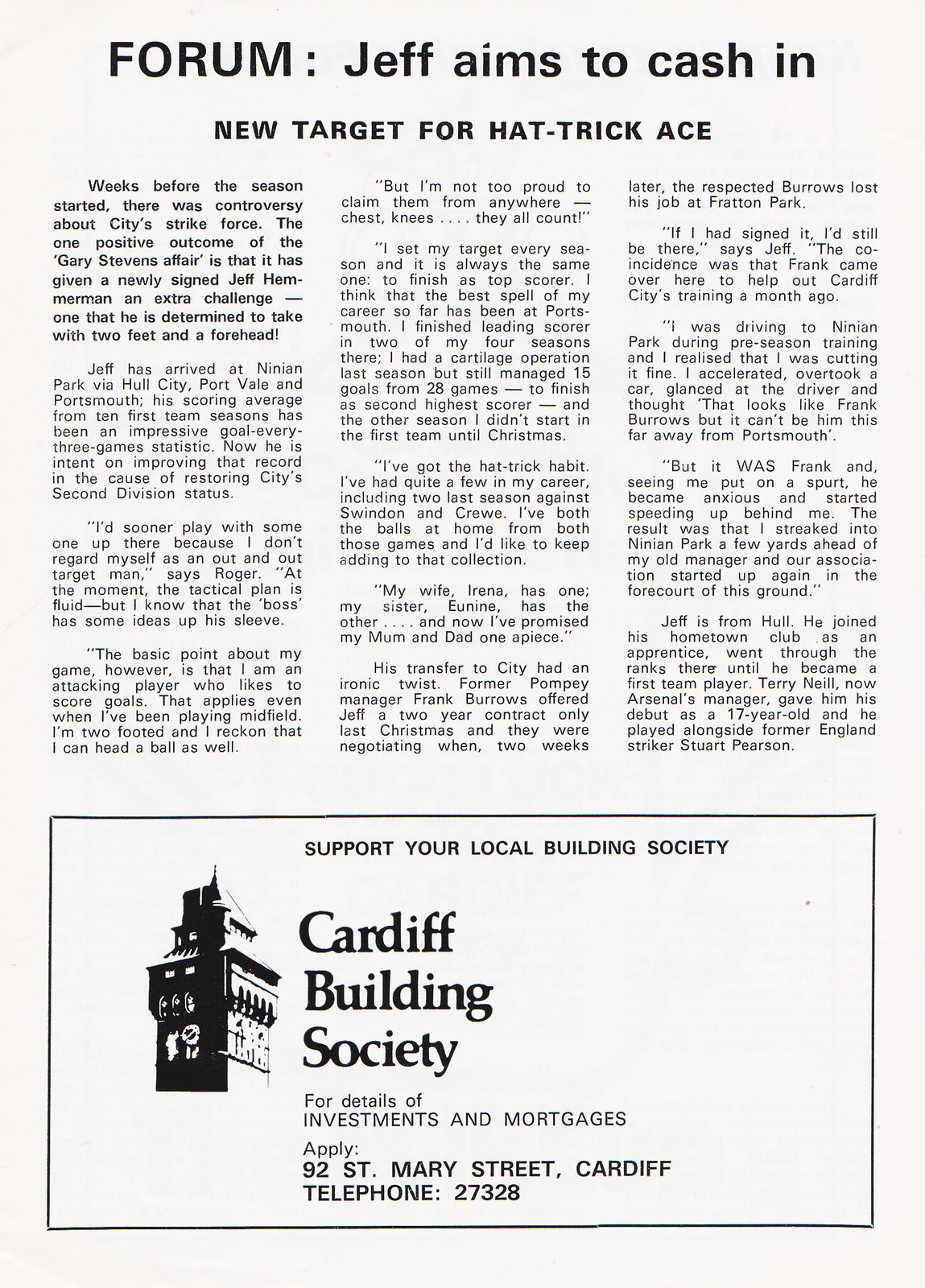The image depicts a page seemingly taken from a magazine or newspaper, under the heading "Forum." The prominent title reads "Jeff aims to cash in," followed by "New target for Hat Trick Ace." The article beneath this title spans about ten paragraphs, divided into three columns. The initial paragraph is bolded and notes, "Weeks before the season started, there was controversy about city strike force. The one positive outcome of the Gary Stevens affair is that it has given a newly signed Jeff Hemmerman an extra challenge. One that he is determined to take with two feet and a forehead." At the bottom of the page, there's a banner advertisement promoting the Cardiff Building Society, urging readers to "Support your local building society." It includes an image of a tower and provides details for investments and mortgages, directing applicants to "Apply, 92 St. Mary Street, Cardiff," and lists a telephone number, 27328. The overall layout and the content suggest a focus on sports, particularly around a notable player, Jeff Hemmerman, and his upcoming challenges.